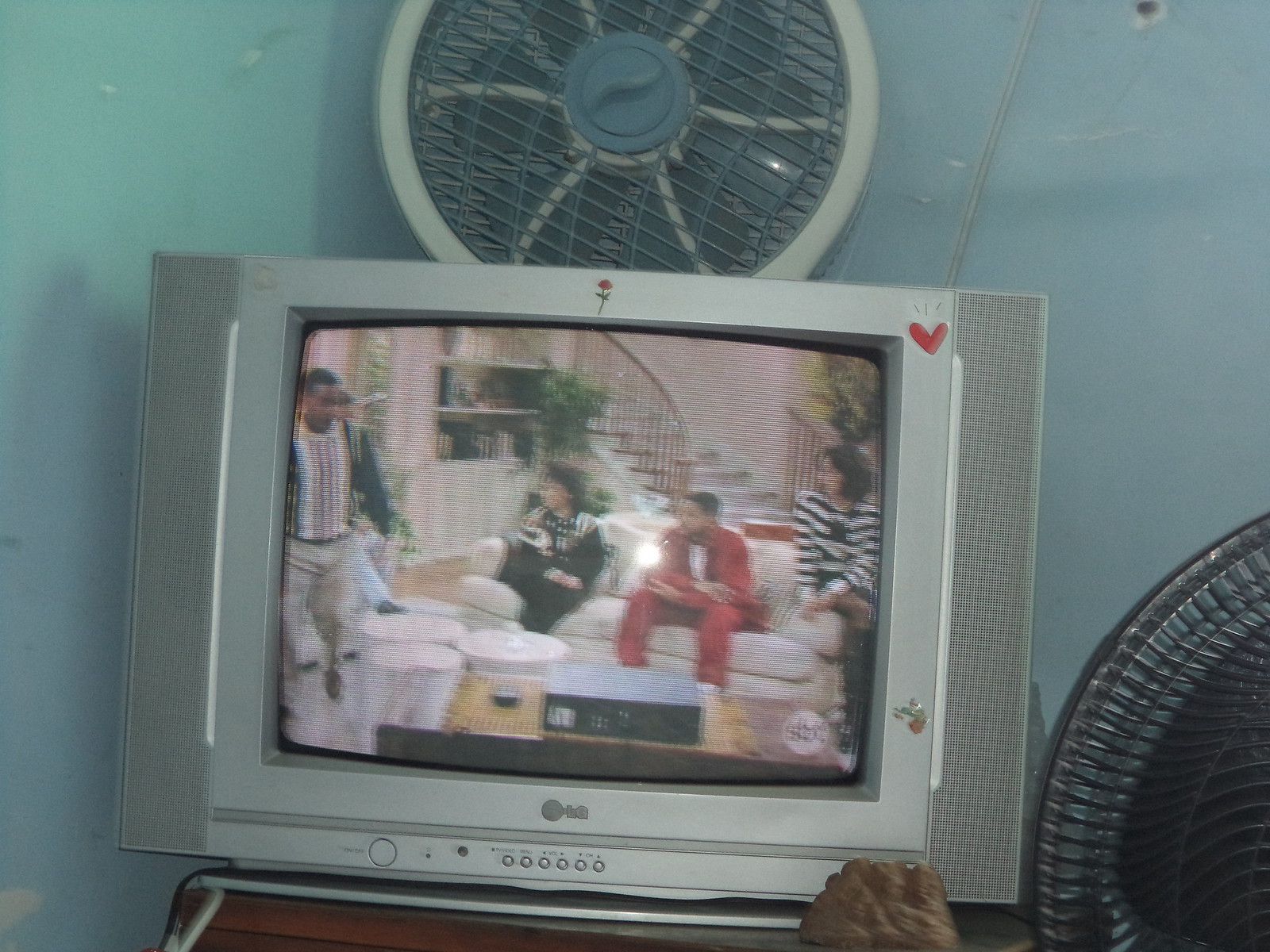The photograph captures an old-school, gray or silver television set from the 90s, approximately 24 inches in size. The television is located atop a brown dresser, though only the top part of the dresser is visible. On the screen, an episode of "The Fresh Prince of Bel-Air" is playing, showing three cast members sitting on a white couch in conversation. Surrounding the scene on the TV, there are several details: a red heart sticker in the top right corner, and a red rose sticker above the screen. The TV has built-in speakers on either side and appears to be an LG model. Atop the television, there are two round mechanical fans, one white and one black. The room's wall behind the TV is painted a light blue color, providing a soft backdrop. In the lower right-hand corner, a black-toned hand is visible, seemingly enjoying the show. The overall image is well-lit with natural light, making all elements and colors distinct.